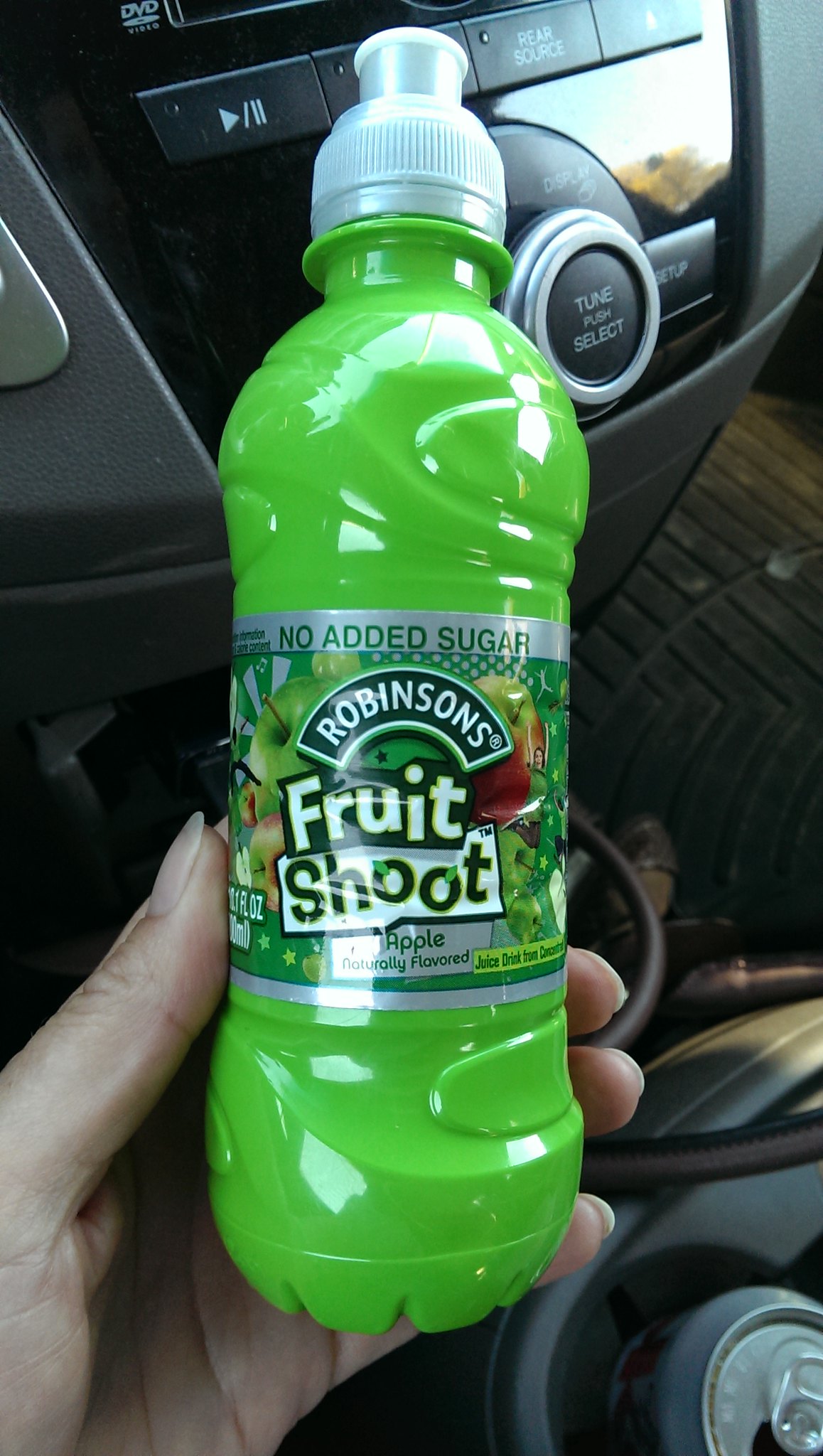In this photograph, we see a woman's hand, with neatly done nails, holding a lime green plastic bottle of Robinson's Fruit Shoot inside a car. The bottle, with a gray screw-on cap featuring a white pop-up section for resealing, prominently displays text indicating "No Sugar Added," "Apple," and "Naturally Flavored." The label is affixed to a flat area of the bottle flanked by bulbous, textured sections. Behind the hand, the car’s center dashboard is visible, featuring controls including a "tune, push to select" button and DVD functions. In the center console, a drink holder contains an open soda can, and cables are looped around the floor mats. The hand's thumb is positioned on the left side of the bottle, with the last three fingers peeking around the edge.